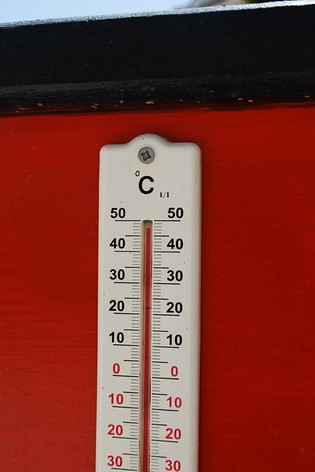Close-up of a room thermometer mounted against a vivid red background, which could either be a wall or a cabinet. The red surface is accentuated by a black-painted trim at the top. The thermometer features a sleek white casing, displaying temperature readings in degrees Celsius, as indicated by the letter 'C' above the numerals. Temperature ranges are color-coded: from -30 to 0 degrees in red and from 10 to 50 degrees in blue. The red mercury inside the thermometer has ascended to the 48-degree mark, indicating a current temperature of 48 degrees Celsius.